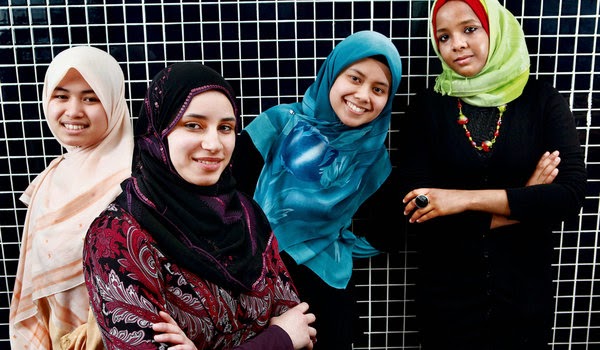In the image, four women are posing together in front of a black wall adorned with a striking white crisscross pattern. Each woman is wearing a distinctive headscarf, adding vibrant splashes of color to the scene. Starting from the left, the first woman with medium-toned skin is adorned in a light pastel pink headscarf with darker pink accents. Next to her stands a lighter-skinned woman, her arms crossed behind her, wearing a black headscarf with purple piping and a floral-printed dark red and black and white shirt. The third woman, also lighter-skinned, dons a bright blue headdress and wears a black outfit. Finally, the woman on the far right, who has darker skin, is distinguished by her bright green headscarf with red piping, black outfit, and a colorful necklace. Each of the women has brunette hair beneath their headscarves, and two of them have their arms crossed.